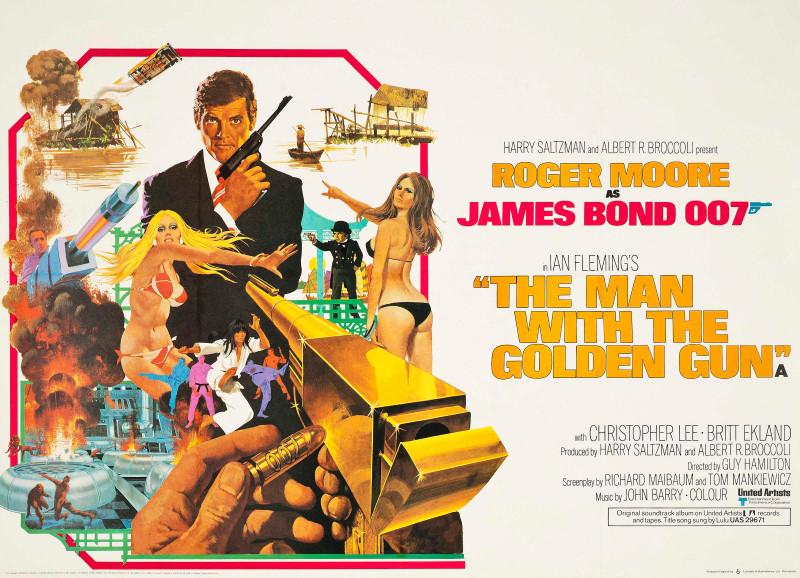This horizontal movie poster advertises the famous James Bond film "The Man with the Golden Gun," set against a grayish-white background. The left side of the poster features a complex and busy illustration, anchored by James Bond, played by Roger Moore, centrally positioned with a black Ruger pistol in hand and outlined in red. Surrounding him in vivid detail, there is a golden gun aimed at him, with a golden bullet marked "007" being loaded into it. The chaotic scene includes a house explosion at the top, a rocket launching beneath it, a fierce fire, and a male hand gripping a bullet. Scantily-clad women in bikinis are placed throughout, a boat scene is depicted above, and karate fighters in action add to the dynamic atmosphere. The right side of the poster displays informative text: "Roger Moore as James Bond 007" and "Ian Fleming's The Man with the Golden Gun," followed by the film's credits listing notable figures such as producers Harry Saltzman and Albert R. Broccoli, director Guy Hamilton, screenwriters Richard Maibaum and Tom Mankiewicz, music by John Barry, with the film released by United Artists. The detailed clash of imagery on the poster encapsulates the action-packed essence of the film.